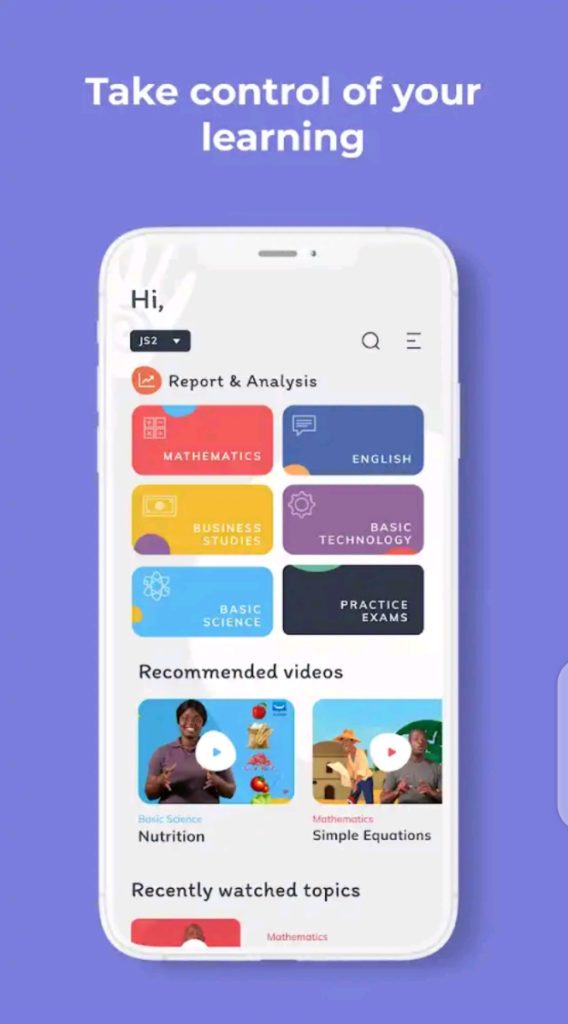On a purple-blue gradient background, the image features the phrase "Take Control of Your Learning" prominently at the top. Centered below is an illustration of a smartphone. On the left side of the phone’s screen, partially obscured by a background handprint, the text "Hi" is displayed, possibly followed by "J52" or "JS2". To the right of this text, there's an icon of a magnifying glass and a sequence of alternating long and short lines.

In the upper right corner of the phone’s screen, the letters "AL" are shown with an arrow extending upwards and to the right. Below, the screen displays various study subjects: Reports and Analytics, Mathematics, English, Business Studies, Basic Technologies, Basic Science, and Practice Exams.

Further below on the phone’s screen is a section labeled "Recommended Videos." One video thumbnail features a lady with black skin, brown hair, and a purple shirt, accompanied by several small icons on the blue background surrounding her. A play button icon overlaps her right shoulder (which is her left from the viewer’s perspective).

Near the bottom of the phone's display, there are topics such as Nutrition and Recent Watch Topics. Another person with black skin, wearing what seems to be a white and black shirt, is pictured, although their attire is harder to discern clearly.